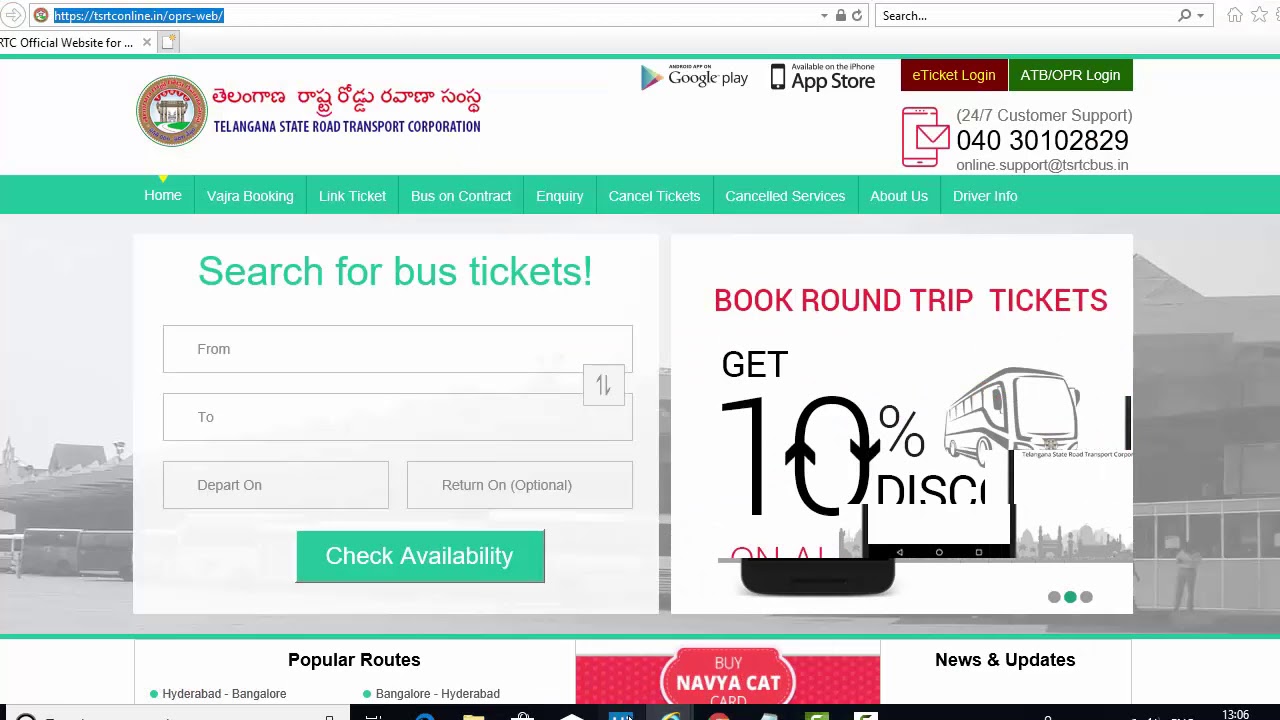This image depicts a website dedicated to bus ticket booking, likely for the Telangana State Road Transport Corporation (TSRTC) in India. The website address at the top is highlighted in blue and unreadable. To its right, there is a search field, along with a home button and a star button. Below this section, it says "RTC Official Website" in one of the tabs.

Text on the page appears to be in an Asian script, possibly Vietnamese, Thai, or Hindi. The main heading reads "Telangana State Road Transport Corporation." Icons for the Google Play Store and Apple App Store are prominently displayed. Nearby tabs include "e-Ticket" and "ATB OPR Login." To the right, a phone number for 24/7 customer service is listed as 040-301-0829, along with icons for a cell phone and an envelope, indicating online support at tsrtcbus.in.

The website's menu options include Home, Varsha Booking, Link Ticket, Bus on Contact, Inquiry, Cancel Tickets, Cancel Services, About Us, Driver & Co., Info. The currently selected menu item is highlighted in green, which is "Home." Below this is a section with the header "Search for Bus Tickets!" followed by input fields labeled From, To, Depart on, Return on—all of which are optional and currently unselected. A green button labeled "Check Availability" is positioned to the right.

Next to the availability check button, there’s a red text offering, "Book round-trip tickets and get 10% discount." This section has a graphic of a bus against a city skyline background. These elements overlap a black and white image that appears to portray a bus terminal, though it's ambiguous whether it's a photograph or a graphic.

Towards the bottom of the image, partially obscured by the desktop taskbar, are sections labeled "Popular Routes," "Buy a Via Card," and "News & Updates."